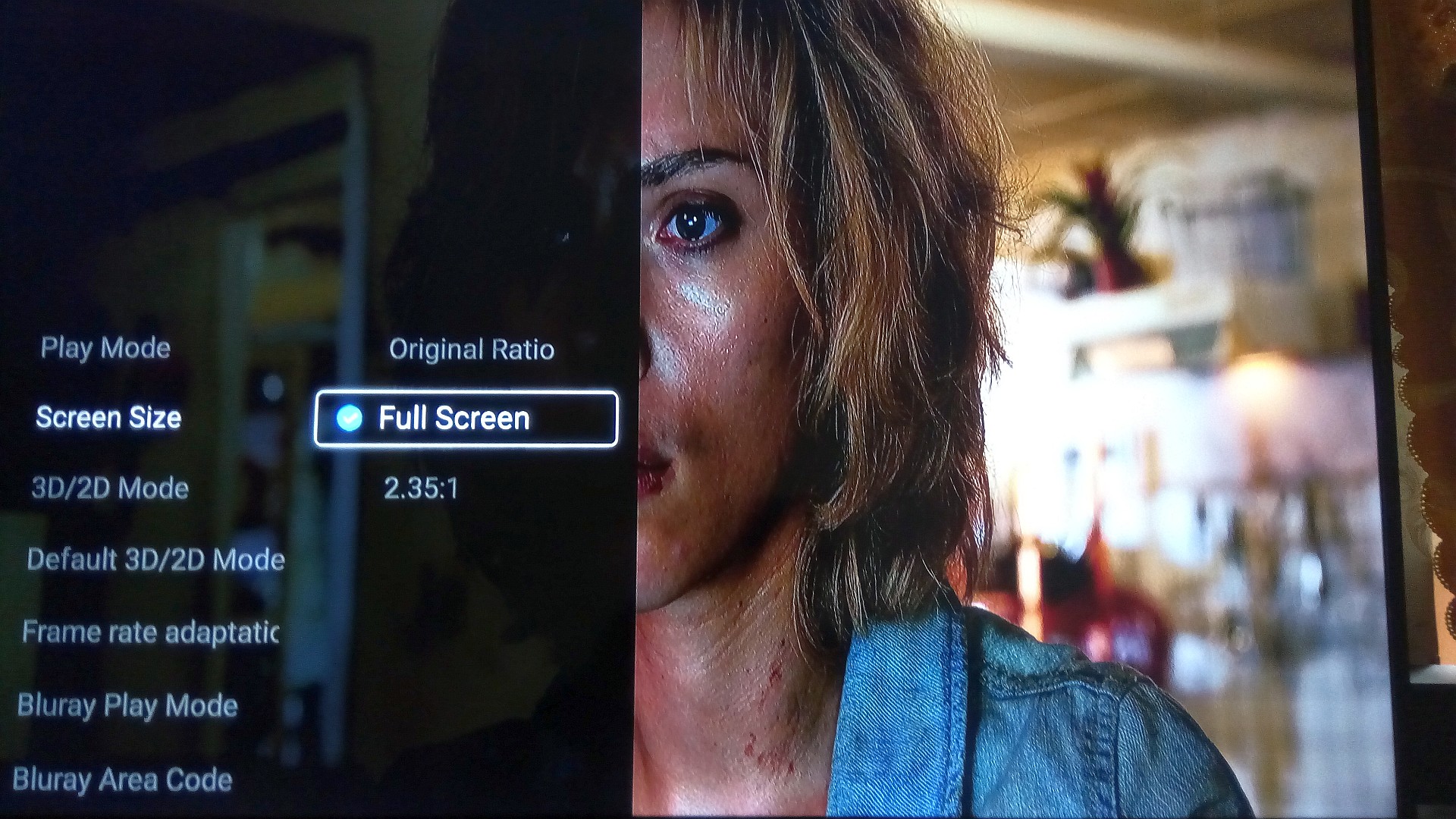The image depicts a paused movie screen showing a split view. On the left half, there is a black menu screen with white text organized into two columns. The left column lists various playback settings: "Play Mode," "Screen Size," "3D/2D Mode," "Default 3D/2D Mode," "Frame Rate Adaptive," "Blu-ray Play Mode," and "Blu-ray Area Code." The right column options include "Original Ratio," "Full Screen," and "2.35:1."

The right half of the screen reveals a close-up of actress Scarlett Johansson, identifiable by her facial features and blonde hair. Her gaze is directed off-camera, and she appears to be in a tense situation, with visible blood or a bruise on her neck, and sweat adding a sheen to her tanned skin. She is dressed in a denim shirt, and the background is blurred, possibly indicating a store or large open space. The image clearly captures the contrast between the active menu settings on the left and Johansson's intense expression on the right.